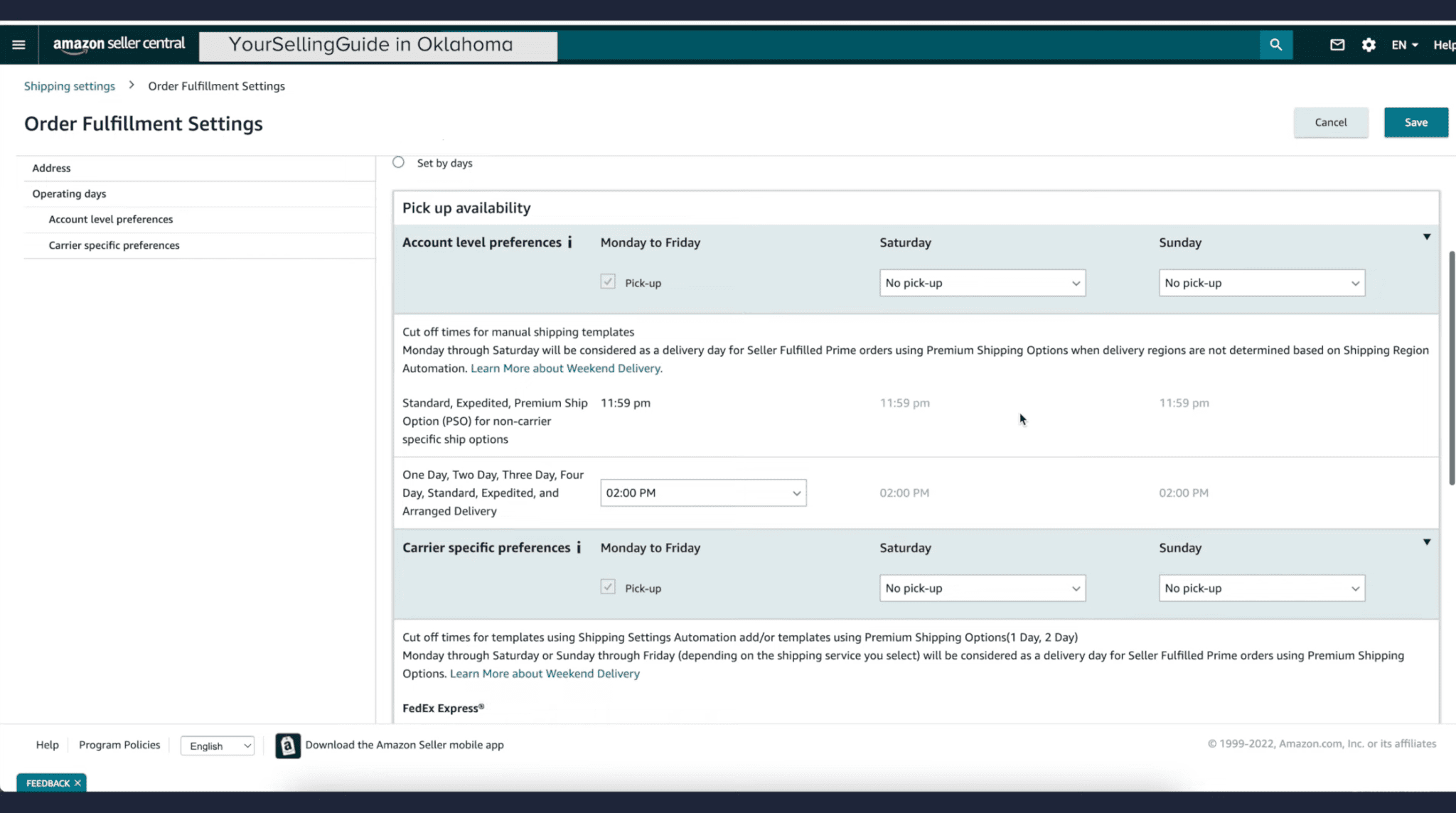Here is a polished and descriptive caption based on the provided information:

---

This image showcases a screenshot of the Amazon Seller Central website interface. The layout features a cohesive design with dark blue horizontal bars along the top and bottom edges of the screen. At the top, a menu bar contains a distinctive icon with three horizontal lines on the left, next to the white text "Amazon Seller Central" set against a lighter blue background.

Centrally positioned across the top is a search bar. The search bar's leftmost portion is a white rectangle displaying the placeholder text "Your Selling Guide in Oklahoma." Adjacent to this, the rest of the search bar is blue, featuring a lighter blue rectangle with a magnifying glass icon.

To the immediate left of the search bar are icons for messages, settings, and language preferences. A slightly cut-off "Help" option is also visible in this area. The main background of the page is white, providing a clean backdrop for the interface content.

Dominating the main content area, the page title "Shipping Settings" appears in blue, followed by a breadcrumb trail indicated by the greater-than symbol leading to "Order Fulfillment Settings." Below this title, a header labeled "Order Fulfillment Settings" is present.

On the left side of the page, a menu lists options such as "Access," "Operating Days," and "Account Level Preferences." On the right, there are several drop-down menus for configuring days, times, and carrier-specific preferences. These menus are styled in lighter blue with white drop-down options, maintaining symmetry and ease of navigation throughout the interface.

The overall design is simple, intuitive, and user-friendly, ensuring that sellers can efficiently manage their orders and shipping settings.

---

This caption offers a clear and meticulous description of the visual and functional elements of the Amazon Seller Central website interface.